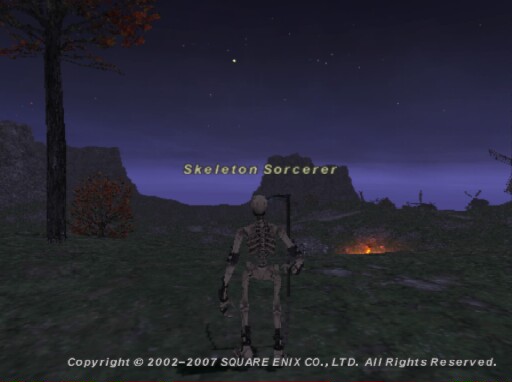This image is a low-resolution, blurry screenshot of a graphical artwork from a video game, likely from the early 2000s. The scene appears to be set in an outdoor environment under a dark blue sky that transitions to black, dotted with faint stars. In the midground, there is an open fire, possibly a campfire. To the left, there's a tall tree with red or orange leaves next to a bush with similar foliage. The ground is green and rocky, with some grassy textures. In the background, rocky cliffs or outcroppings rise toward the horizon. Central to the image is the back of a skeleton figure, reminiscent of the Grim Reaper, holding a scythe. Above this figure, in yellow text, it says "Skeleton Sorcerer." At the bottom of the image, in white text, it reads, "Copyright 2002-2007 Square Enix Co., Ltd. All Rights Reserved."